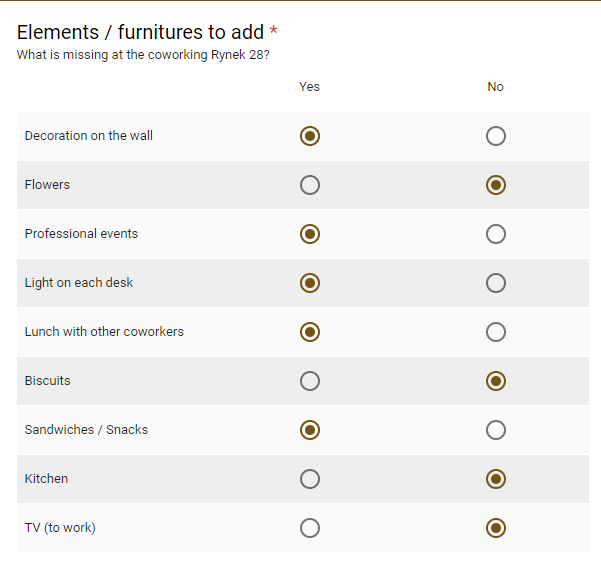This is a vertical rectangular image with the longer side extending from top to bottom. A thin black horizontal line runs across the very top of the image. Directly below this line, there is text that reads, "Elements/Furnitures to add *" followed by the question, "What is missing at the co-working Rhineck 28?" 

Beneath this text, the image features two columns labeled "Yes" and "No." Along the left side of the image, there are various labels listed vertically, each relating to different elements or furnishings typically found in a co-working space. The specific labels and their corresponding answers are as follows:

1. Decoration on the wall - Yes
2. Flowers - No
3. Professional events - Yes
4. Light on each desk - Yes
5. Lunch with other co-workers - Yes
6. Biscuits - No
7. Sandwiches/Snacks - Yes
8. Kitchen - No
9. TV to work - No

These labels and answers are presented in alternating row colors, creating a striped pattern. The first row, "Decoration on the wall," has an off-white background, while the second row, "Flowers," has a light gray background. This pattern continues to alternate down the list, helping to visually distinguish each item.

Overall, the image is a detailed checklist intended to identify the current features and missing elements at the co-working space Rhineck 28.